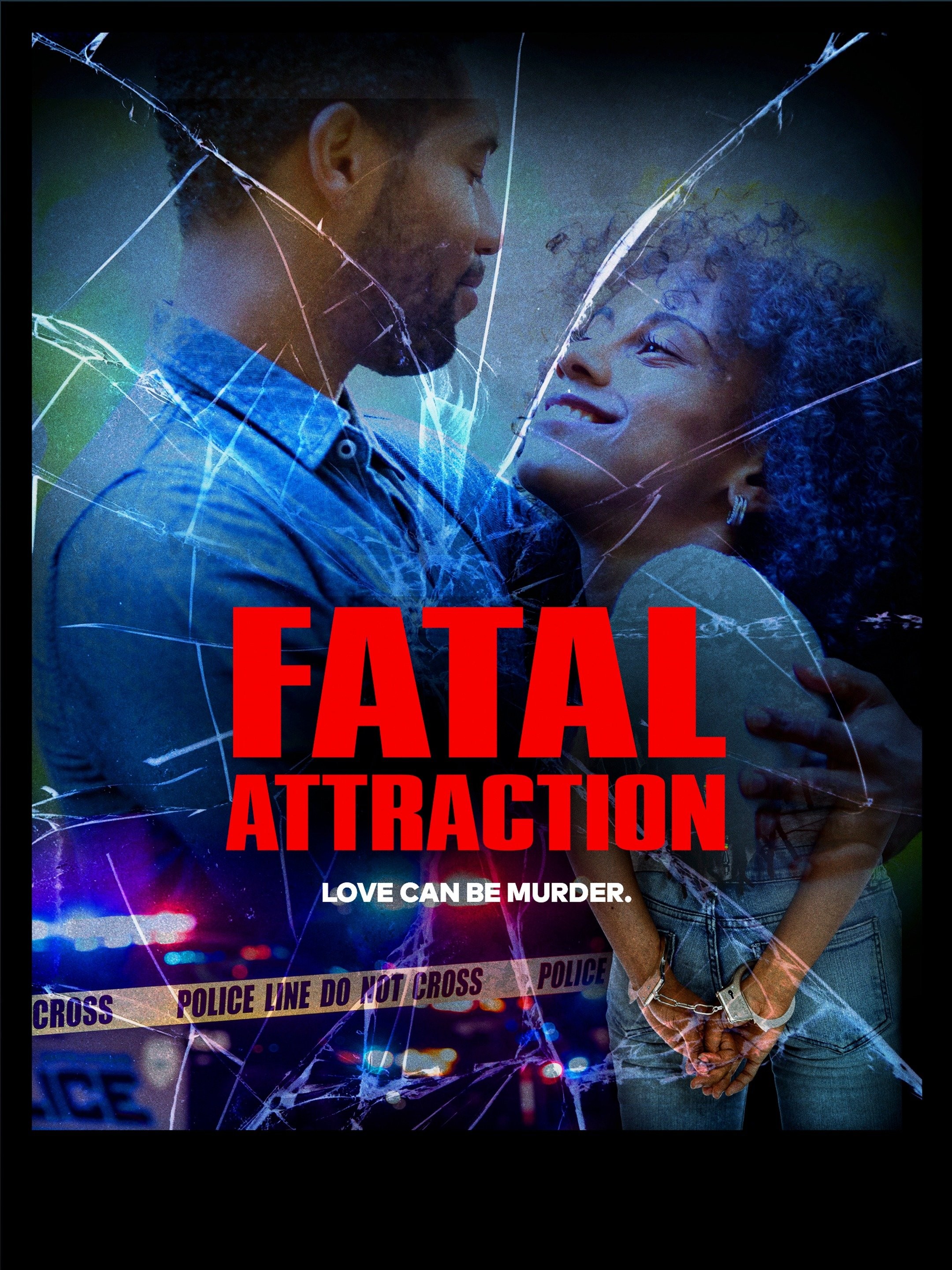The movie poster prominently features the title "FATAL ATTRACTION" in bold, red, all-capital letters, which appears to be in an impact font. Below the title, in smaller white, all-capital letters, is the tagline "LOVE CAN BE MURDER." The background consists of a collage with distinct elements: a couple looking into each other's eyes, both depicted as black individuals, with the man on the left and the woman on the right. The entire image is overlaid with a cracked glass effect, adding a sense of tension and violence. Below the tagline is yellow police line tape that reads "POLICE LINE DO NOT CROSS," adding to the ominous atmosphere. At the bottom left of the image, there is a depiction of a police car's siren, while on the bottom right, there are hands in handcuffs, indicating an arrest. The overall design suggests a theme of crime and dangerous romance, captured with a nostalgic yet intense visual style.